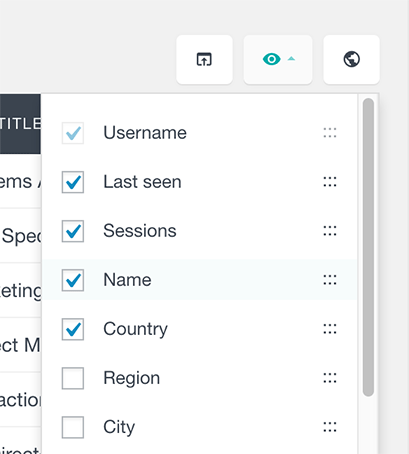This image depicts a webpage displaying user account details. The text entries on the page include "Username", "Last Seen", "Sessions", "Name", "Country", "Region", and "City". Among these, "Username", "Last Seen", "Sessions", "Name", and "Country" are marked with checkmarks, indicating selection or confirmation, whereas "Region" and "City" are not checked. At the top of the page, icons for view, share, and web functions are visible. To the right of the image, a vertical scroll bar is present, suggesting that more information is available by scrolling. The color scheme primarily consists of blue and black elements set against a white background, providing a clean and professional appearance. Additionally, the left pane contains text, although some portions are obscured, rendering them partially unreadable.